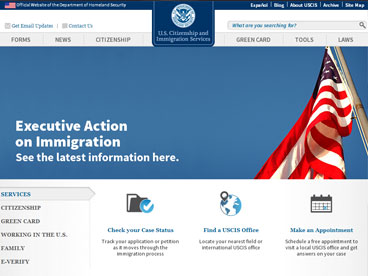This image features a webpage from the U.S. Citizenship and Immigration Services (USCIS). Dominating the page is a large, blue box highlighting the phrase "Executive Action on Immigration" in white text. The box invites users to "See the latest information here." Above the text is a dynamic photograph of an American flag, captured from a low angle, fluttering against the sky.

The top navigation bar of the website offers various categories, including "Forms," "News," "Citizenship," "Green Card," "Tools," and "Laws." Each category appears to have dropdown menus containing further options, such as "Family," "Working in the U.S.," and "Green Card." The webpage also provides functionalities to "Check your status," "Find an office," and "Make an appointment," which are essential tools for individuals navigating the immigration process.

At the top left corner, the website bears the official heading of "U.S. Citizenship and Immigration Services," indicating that it is an authoritative resource for immigrants seeking citizenship or other forms of residency in the United States.